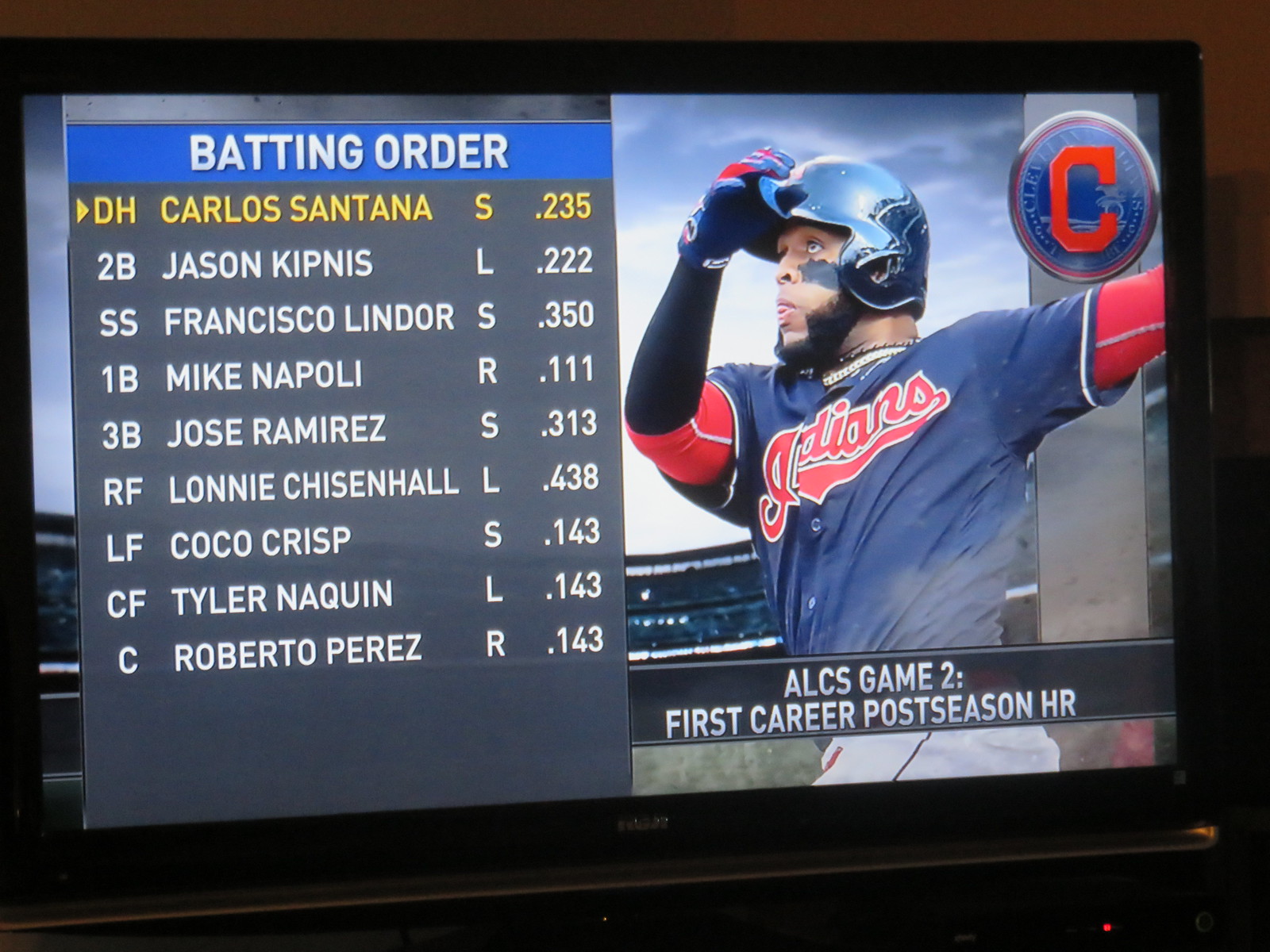The image is a rectangular horizontal photograph, capturing a graphic displayed on a television screen during a Cleveland Indians baseball game. The background is mostly black with a strip of sky visible above the graphic, suggesting it replicates a stadium scoreboard or billboard. On the left side, there is a slate blue surface with a bright blue banner at the top that reads "BATTING ORDER" in white capital letters. Below this header, the batting lineup is listed, detailing the players' positions, names, batting averages, and hitting styles. The player currently at bat is highlighted in yellow. 

The lineup is as follows:
1. DH Carlos Santana (.235)
2. 2B Jason Kipnis (.222)
3. SS Francisco Lindor (.350)
4. 1B Mike Napoli (.111)
5. 3B Jose Ramirez (.313)
6. RF Lonnie Chisenhall (.438)
7. LF Coco Crisp (.143)
8. CF Tyler Naquin (.143)
9. C Roberto Perez (.130)

On the right side of the screen, there is an image of a player in the midst of a swing, attired in a blue Cleveland Indians jersey with red and dark sleeves underneath, and wearing a batting helmet. His left arm is holding the helmet, and though his right arm is only visible up to the elbow, it presumably holds the bat. There is a prominent red 'C' in a circle near the corner of this image, and text below it reads "ALCS Game 2, First Career Postseason HR." This scene vividly portrays the intensity and excitement surrounding the player's moment at bat during the game.